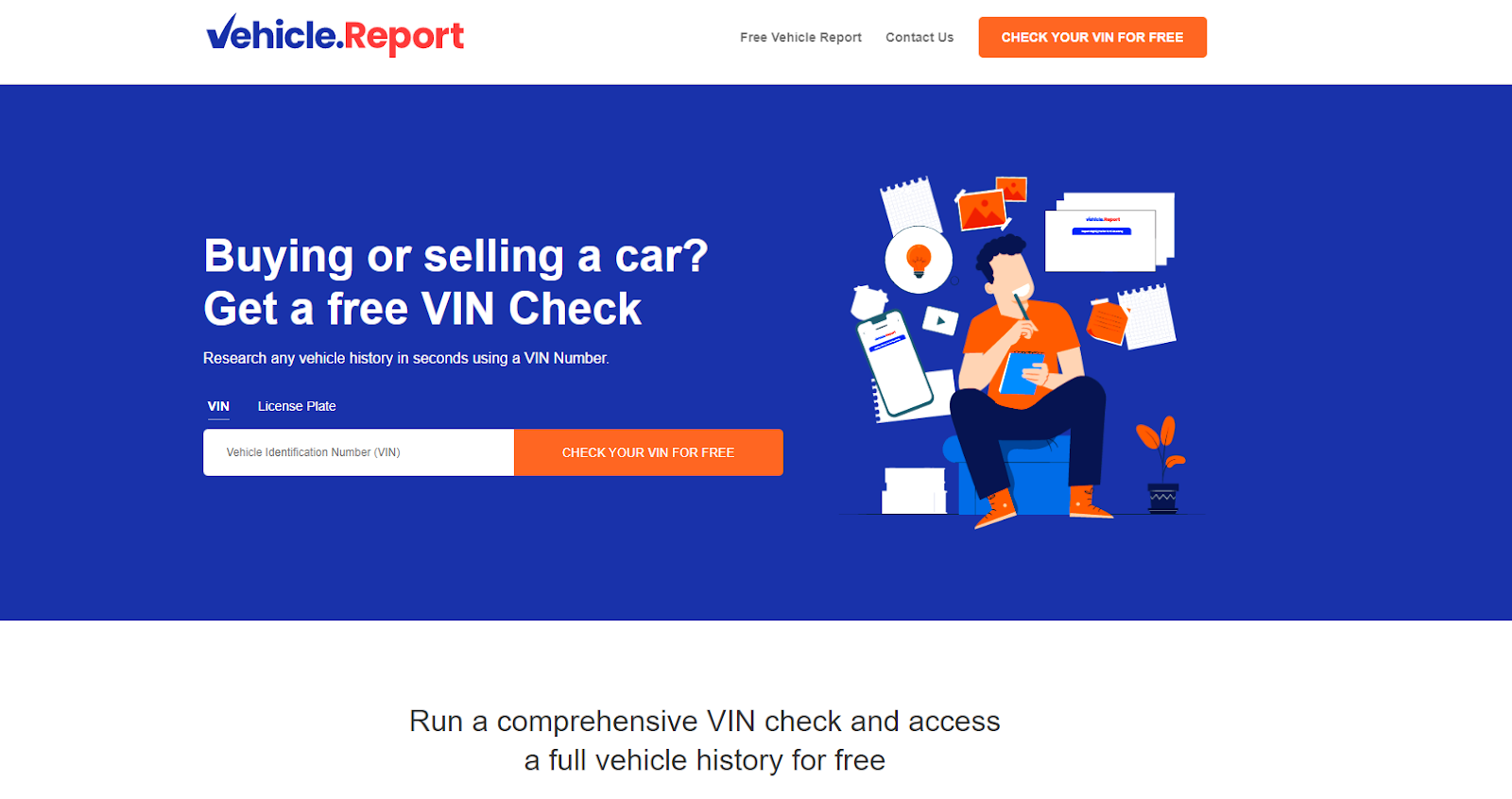The image displays a webpage with a predominantly white background accented by blue, red, and orange elements. At the top of the page, there is a blue logo featuring the word "Vehicle," where the "V" is stylized as a checkmark, followed by the word "Report" written in red. The phrase “Vehicle Report” appears again, possibly in an orange hue. 

There are several tabs at the top of the page, including one labeled "Free Vehicle Report" and another that says "Contact Us." A prominent orange rectangular button with white text reads "Check Your VIN for Free."

The main page has a blue background. On the left side, a message encourages buying or selling a car with a free VIN check. It mentions that users can research any vehicle's history in seconds using a Vehicle Identification Number (VIN). The dropdown menu has "VIN" selected, and an orange button again states "Check Your VIN for Free."

A cartoon graphic is displayed featuring a man sitting on a blue chair. The man is holding a pencil up to his mouth and a tablet in his hand, though his facial features are not visible; only his dark hair is shown. Next to him is a potted plant with orange leaves, also rendered in a cartoon style.